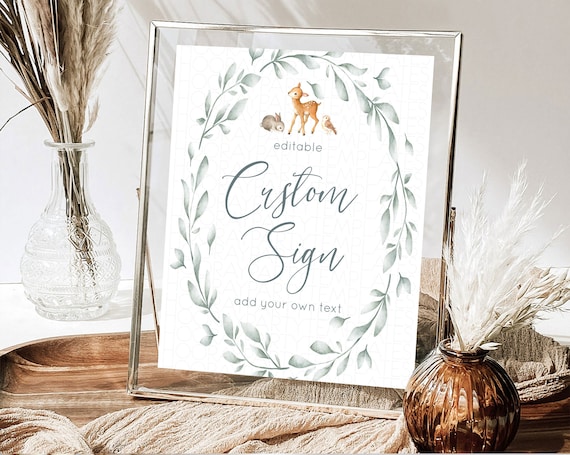The image appears to be an advertisement for customizable signs, possibly featured on a website like Etsy that specializes in printing services. The central focus is a sign displayed in a sophisticated glass frame with a thin metal edge. The frame is positioned on a small wooden table draped with a light beige cloth. Centered within the frame is a white background adorned with a watercolor wreath of light gray leaves, and at the top, there's an illustration of a baby deer and a bunny. The text within the frame, rendered in an elegant sage green font, reads "Editable Custom Sign, Add Your Own Text." To the left of the frame stands a clear vase filled with wheat stalks, while to the right, a small brown vase, reminiscent of the bottom of an old-fashioned perfume bottle, contains white wispy plants or branches. The backdrop is a neutral gray wall, complementing the overall aesthetic of the setup.